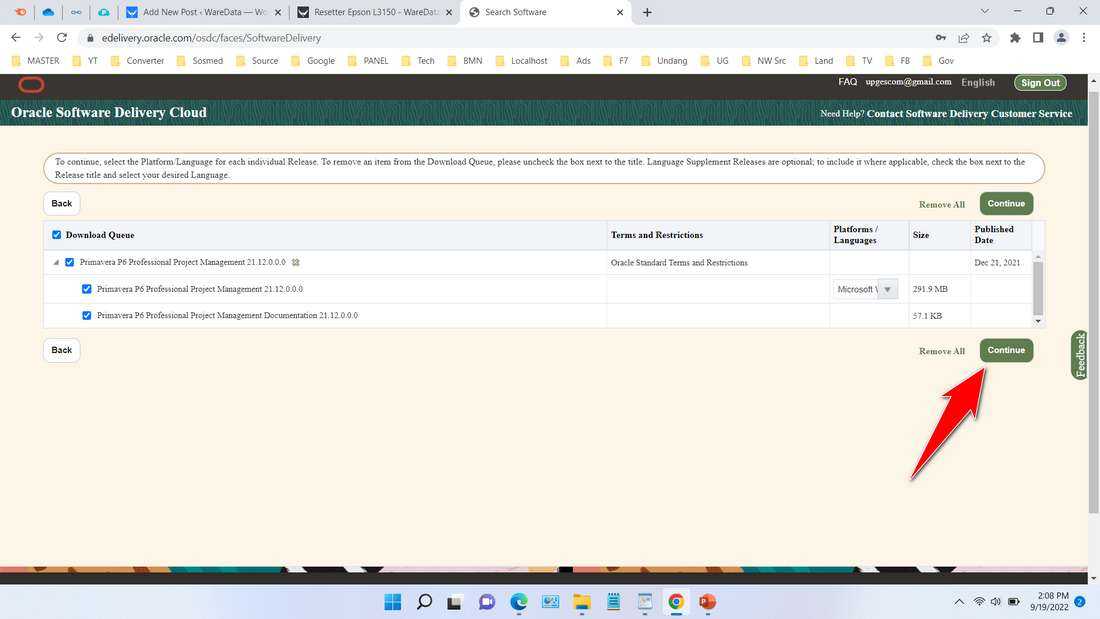A screenshot of a computer screen displaying the Oracle Software Delivery Cloud webpage. At the top right corner of the page, there are navigation options including an "FAQ" link, the logged-in email address (upgericom@gmail.com), a language selection set to English, and a sign-out button. The main section of the screen prominently features the Oracle Software Delivery Cloud logo and a help prompt stating, "Need help? Contact software delivery customer service."

Beneath this header, text instructions explain how to manage the download queue: "To continue, select the platform language for each individual release. To remove an item from the download queue, please uncheck the box next to the title. Language supplement releases are optional. To include where applicable, check the box next to the release title and select your desired language." 

Below the instructions, there is a section that resembles an email inbox, with columns labeled "Download Queue," "Terms and Restrictions," "Platform/Languages," "Size," and "Publish Date." Currently, three items are listed in the download queue, though the specific details are difficult to read. A prominent green continue button with a red arrow pointing towards it is situated at the bottom of this section.